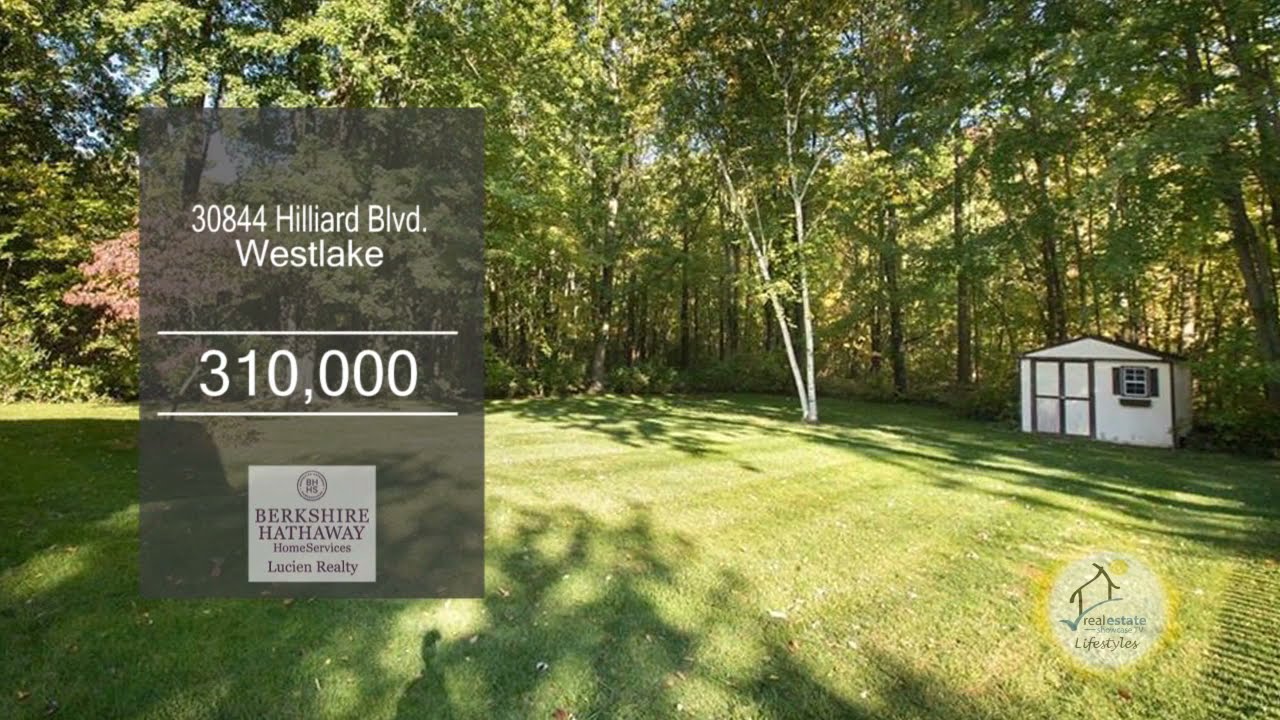This image depicts a spacious, well-kept backyard, featuring a large, grassy area that stretches horizontally across the scene. Tall green trees form a lush backdrop, with patches of blue sky peeking through the upper branches, defining the top boundary of the image. In the middle right section of the yard, near the edge of the wooded area, there is a small white shed with brown or green trim, and a tiny window. On the left side of the image, a faded black vertical rectangle prominently displays text that reads "30844 Hilliard Boulevard, Westlake." Below this, there are horizontal lines separating the price "310,000" and the real estate information "Berkshire Hathaway, Lucien Realty," all written in white. In the bottom right corner of the image, there's a yellow circle with an indistinct symbol and writing. The overall scene captures the tranquility and openness of a residential property listing, accented by clear real estate details.